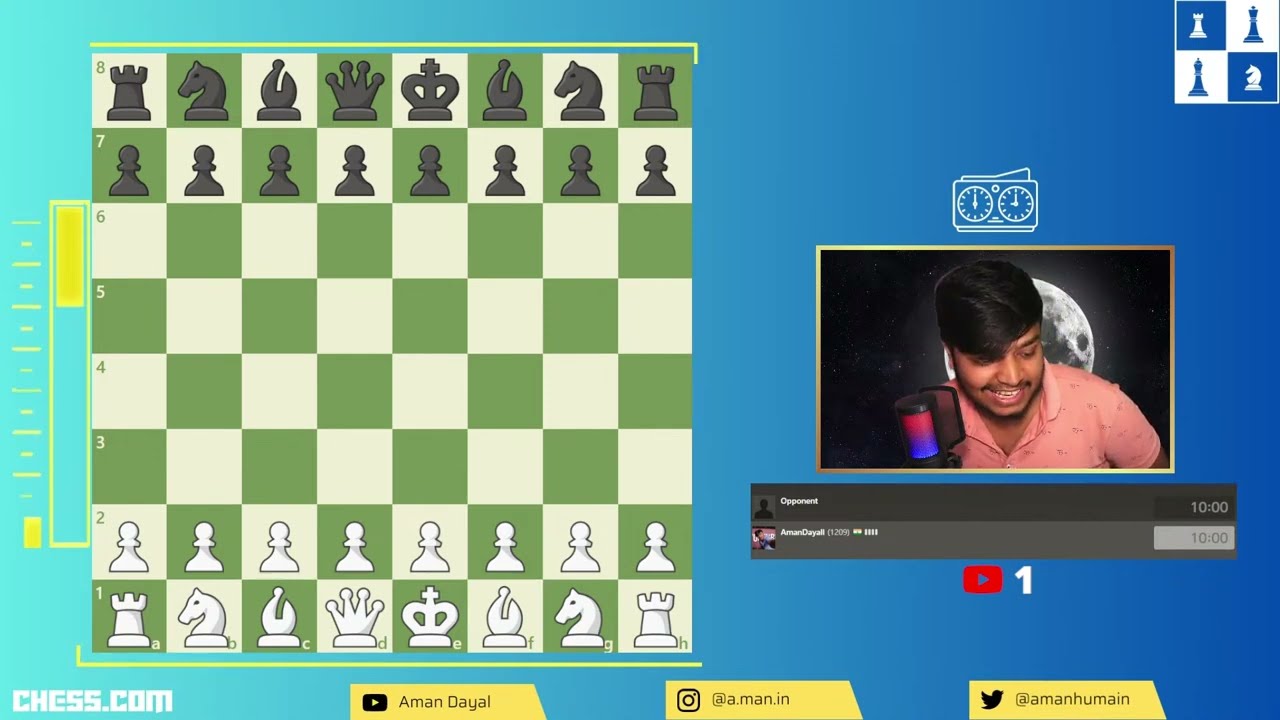The image captures a screen grab of an online chess game streamed on chess.com. The left half of the screen displays a virtual chessboard, positioned at the initial stages of the game with black and white pieces intact on a green and light green checkered background. Text in the bottom left corner reads "chess.com." The right half features an inset video stream of the player, a man with black hair and a beard, wearing a salmon-colored shirt, and speaking into a black, red, and blue microphone. Behind him is a white moon on a gradient blue background that transitions from light blue to dark blue. Above the player’s video is a standard chess clock, and in the top right corner, there is a 2x2 logo featuring various chess pieces. At the bottom of the image are three yellow banners displaying the player’s social media handles: Aman Dayal on YouTube, @a.man.in on Instagram, and @AmanHumane on Twitter. The overall setting suggests that the player is streaming a live chess match, sharing both the game and his commentary simultaneously.